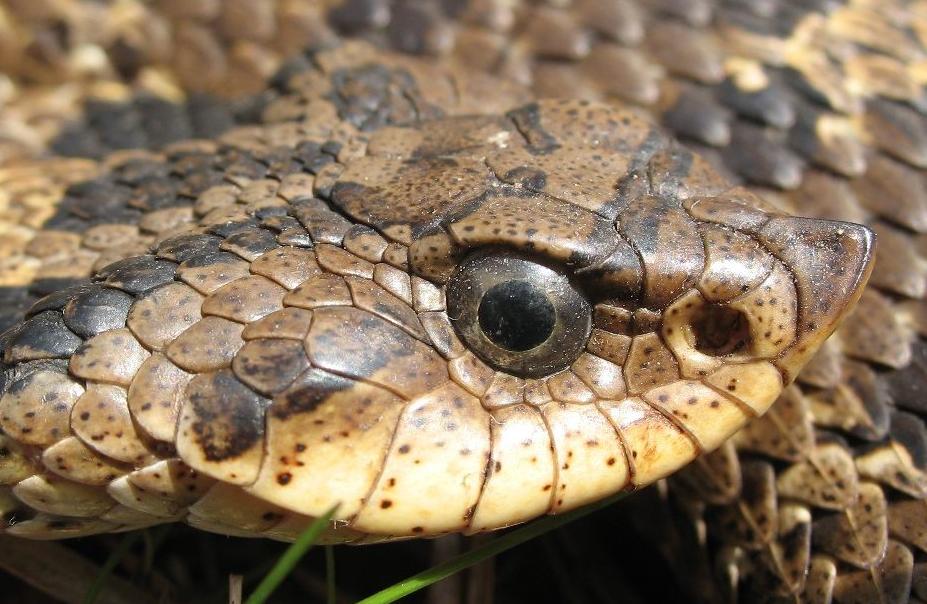The image is a closely zoomed-in, rectangular photograph showcasing the intricacies of a coiled brown snake. The center focal point of the image is the snake's head, particularly emphasizing its brown eye with a black pupil. The snake's nostrils and pointed snout are also clearly visible. The background is composed entirely of the snake's body, displaying an intricate pattern of light yellow, medium brown, to dark brown, and black scales with both spots and striped motifs. Just a couple of small green blades of grass peek through at the bottom of the image, providing the only hint of an external environment. The snake's scales form a textured mosaic, with its tan and speckled face contrasting against the darker, more detailed body that slightly fades as it coils into the background.